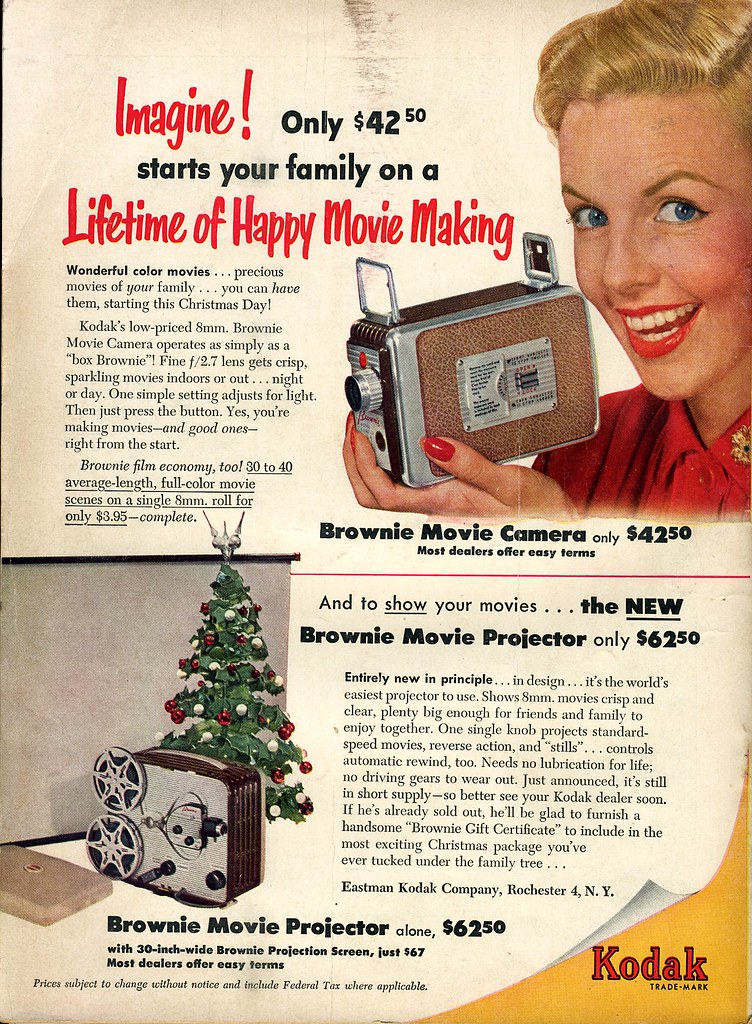This vintage advertisement poster features a nostalgic, aged color scheme and promotes Kodak's Brownie movie cameras and projectors. At the top, in bold red font, it exclaims, "Imagine!" followed by "Only $42.50 starts your family on a lifetime of happy movie making" in black font. A classic, retro-style illustration of a white woman with blue eyes, golden hair, and red lipstick is prominently displayed to the right, holding a vintage camera. Below her, in red font, the text reads, "Brownie movie camera only $42.50." 

On the lower left, there is an old-fashioned movie projector next to a small Christmas tree, labeled "Brownie movie projector." Adjacent to this, it states, "And to show your movies, the new Brownie movie projector only $62.50." Another paragraph of smaller text provides additional details, and the bottom right corner of the poster features the Kodak logo on a yellow background.